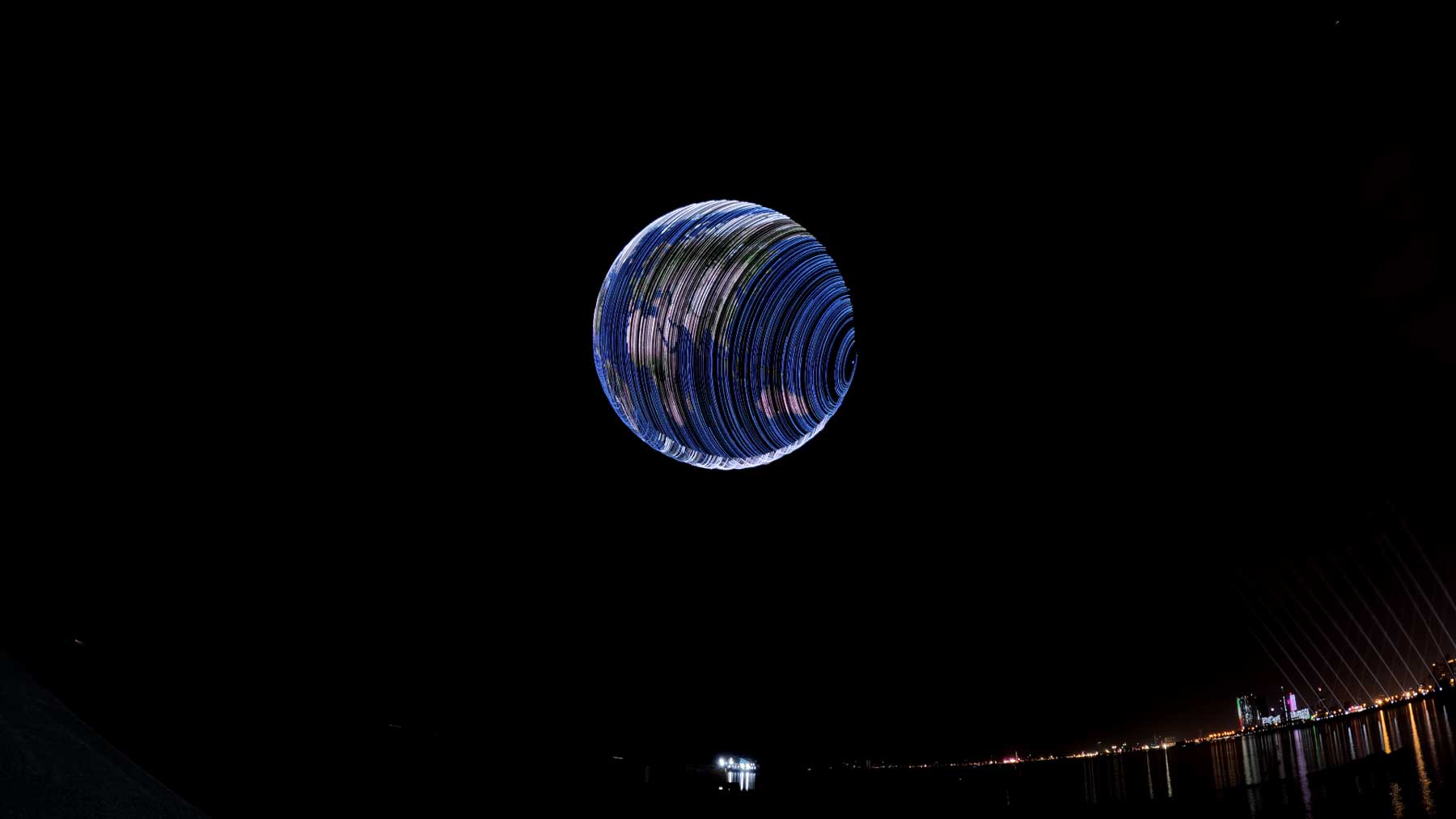The image showcases a surreal nighttime cityscape viewed from across calm waters. The background is pitch-black, creating a stark contrast with the illuminated elements. At the bottom right, a distant city is visible, its skyscrapers and buildings casting a colorful array of lights in white, pink, yellow, orange, green, and red, which are perfectly mirrored in the water below. Dominating the sky is a colossal, glowing blue sphere, seemingly hovering over the city. This sphere, composed of luminescent, circular lines that create an intricate pattern of curved slices, appears to be an abstract or artistic representation of Earth. The continents of Africa, Europe, and Asia are discernible on its surface. The overall feel of the image is otherworldly, blurring the lines between reality and digital manipulation.